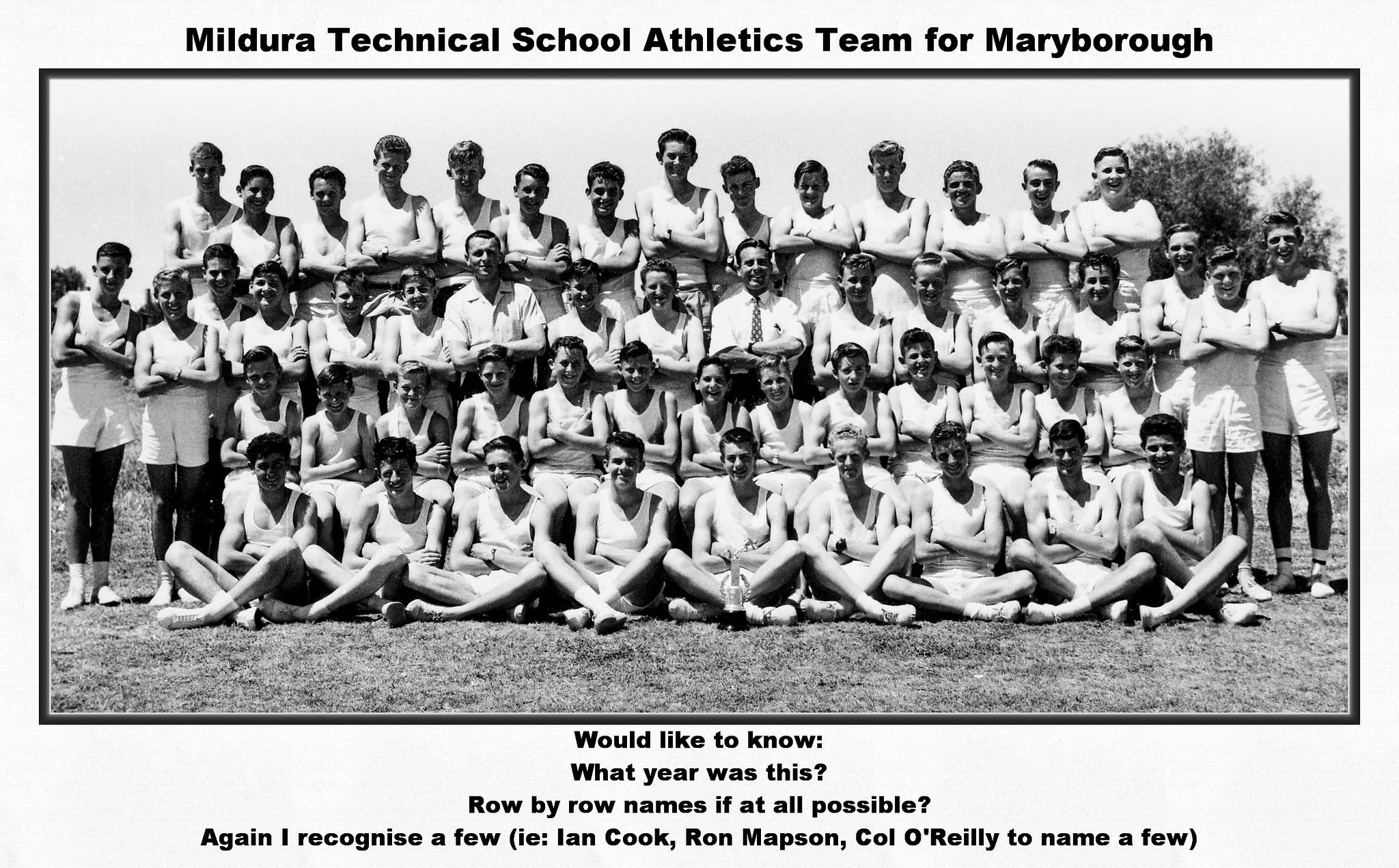The wide rectangular image is framed with a soft gray border, which is thin on the left and right sides but quite thick at the top and bottom. The top border features bold black text that reads, "Mildura Technical School Athletics Team for Maryborough." The bottom border contains text asking for the year and names of the individuals in the photo, mentioning a few recognized names such as Ian Cook, Ron Mapson, and Colonel O'Reilly.

This black and white photograph showcases four rows of young men, presumably part of the athletics team. They are all dressed in white tank tops and white shorts. The layout consists of the bottom row sitting on the ground with their legs crossed, the next row seated on chairs, the third row standing, and the topmost row standing on chairs. One individual in the third row stands out; he is centrally positioned, wearing a white button-down shirt with a tie, rolled-up sleeves, and stands with his arms crossed.

Several of the youths are smiling, while others maintain neutral expressions. The background of the image displays a white sky and a few trees visible at the upper right corner, contributing to the nostalgic atmosphere of this historic team photograph.